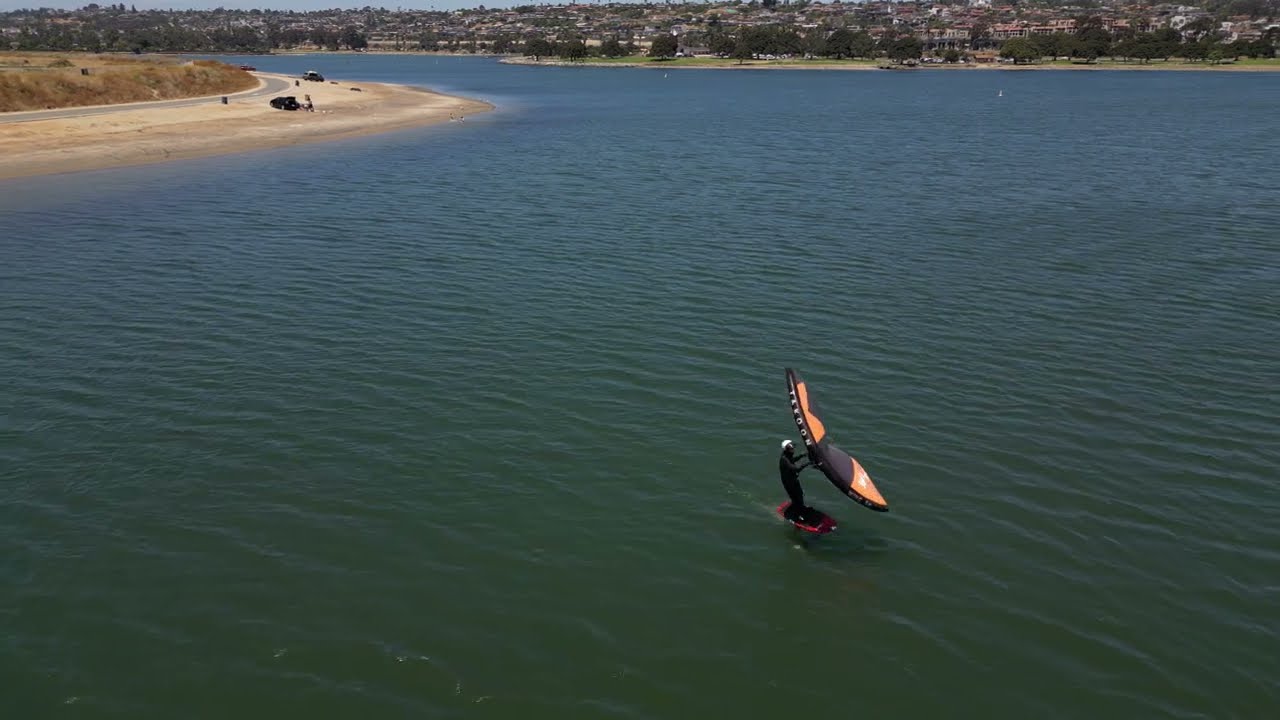The image features a high-angle shot, likely taken from a drone, capturing a scenic waterway that appears to be an inlet or bay near the ocean. The foreground is dominated by a windsurfer on a small surfboard, which is primarily red and black. He is dressed in a black bodysuit and dark clothing with a white helmet or backwards baseball cap. Holding a black and orange sail, the windsurfer is gliding across the greenish-blue water, which has gentle ripples indicating light winds.

To the left of the image, there is a sandy beach outcropping with a few trucks parked and a couple of people fishing in the water. Further in the background, a range of housing developments stretches along the shoreline, characterized by their white facades and red clay-tiled roofs. A road spirals around a grassy hill, and trees are interspersed among the residences, suggesting a high-end suburban area. The overall scene is serene and detailed, highlighting both natural and man-made elements in a harmonious coastal setting.